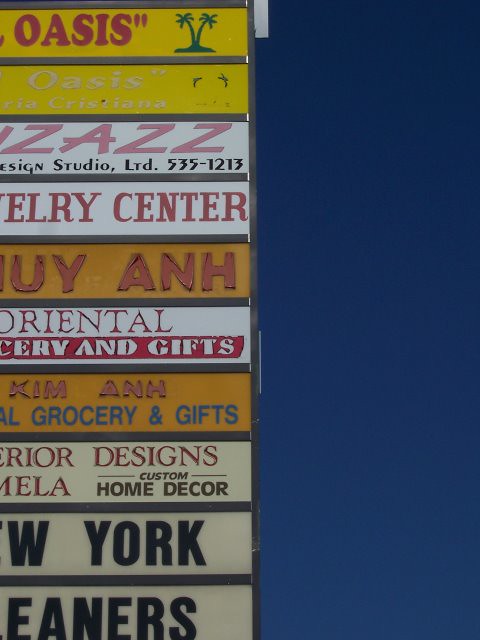This image is divided into two sections. On the left half, there is a series of stacked signs reminiscent of a strip mall or plaza directory near the road, while the right half features a totally clear dark blue strip that might be the sky. The signs on the left vary in shades of yellow, white, and orange backgrounds, with most featuring red lettering, and the bottom two displaying black lettering. There are ten distinct rows listing different businesses, though not all names are fully visible.

From top to bottom, the first sign has a yellow background and reads "Oasis" in red with quotation marks and two green palm trees. The second sign, also on a yellow background, has the word "Oasis" in white. The third sign, against a white background, reads "Zazz Design Studio Limited" along with a telephone number. The fourth row, on a white background, partially shows the word "Jewelry Center", indicated by "E-L-R-Y" and "center". The fifth row has a darker yellow or orange background with red peeling letters that may be non-English, showing "U-Y" and "A-N-H". The sixth sign, on a white background with red letters, reads "Oriental" followed by a red stripe with white letters showing "C-E-R-Y and Gifts". The seventh row has the dark yellow or orange background with peeling red letters "Kim" and "A-N-H", and in blue letters, part of the word "grocery and gifts". The eighth sign, on a white background, displays part of the word "Interior" in red letters ("R-I-O-R") and "Designs", while the second part reads "M-E-L-A" also in red, and "custom home decor" in black letters. The ninth row has a white background and partially displays "New York Cleaners", seen from "W-York". The tenth and bottom sign also on a white background shows a portion of the word "Cleaners" ("E-A-N-E-R-S").

In summary, this photograph features a clear division between a blue strip on the right and a series of colorful, partially visible business signs on the left, typical of a strip mall directory.